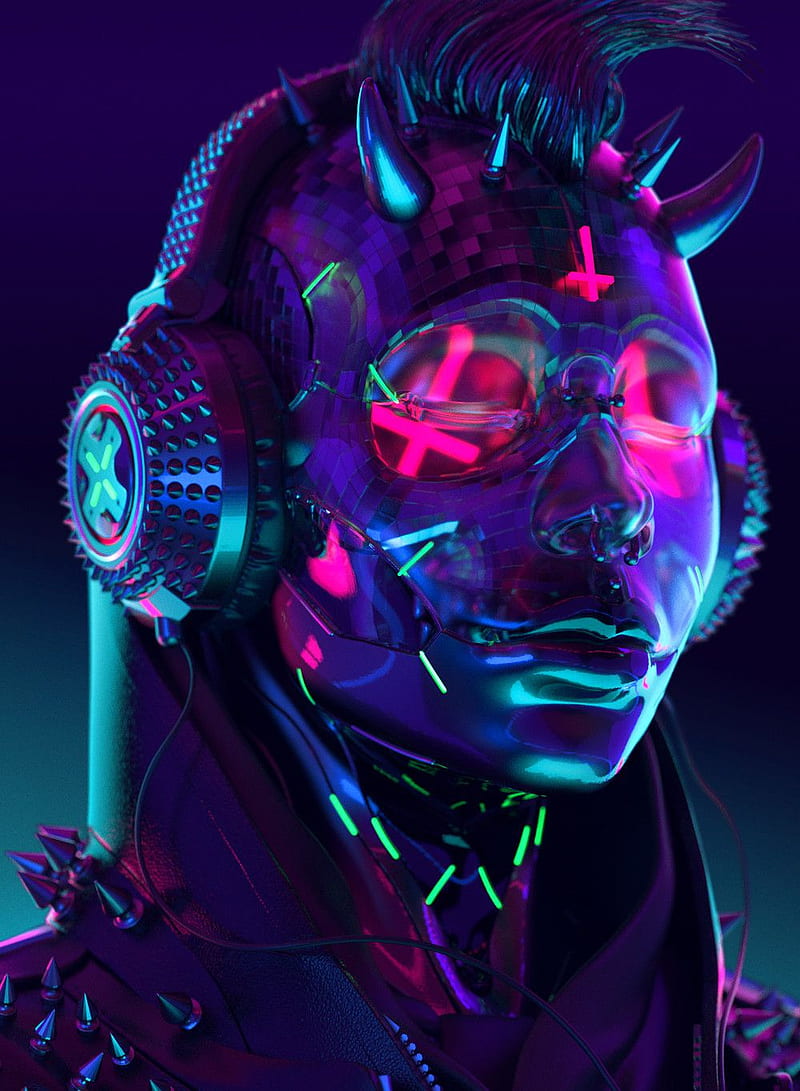This is a computer-generated image of a humanoid figure with a striking, otherworldly appearance. The figure has short hair styled into a mohawk and sports several body modifications including short horns protruding from the scalp. The skin tone of the figure is a captivating chromatic blend of purple, blue, and titanium hues. Its eyes are closed and glasses adorn a face, which exhibits a somber, almost sad expression. 

The figure is wearing a studded hoodie, and a pair of distinctive, spiky headphones that feature a plus-like symbol on the outer center of each ear cup. Radiating from the neck are four slits emitting a vibrant neon glow. Both sides of the headphones are connected with a wire running down from each ear. The composition focuses solely on the head and neck, filling the entire image with dark, atmospheric lighting that emphasizes the surreal, gothic aesthetic. Across the shoulders, barely visible through the darkness, the figure wears what looks like an outfit befitting a goth style. The mouth is closed, adding to the overall melancholy impression.